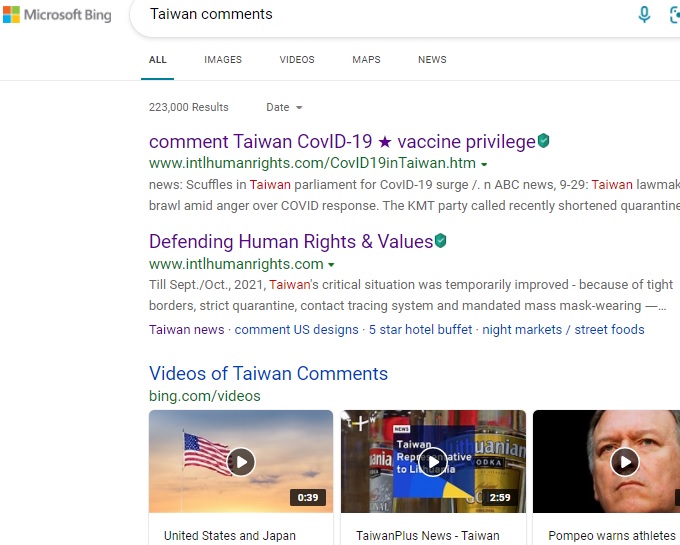Screenshot of a Microsoft Bing search page, captured clearly with distinct features identifiable. In the upper left-hand corner of the webpage, the iconic Microsoft logo is visible, composed of four squares in red, green, blue, and yellow colors arranged together. Adjacent to the logo, the text "Microsoft Bing" is written in a gray font.

Dominating the upper portion of the page is a search bar, within which the phrase "Taiwan comments" has been entered. On the right-hand side of this search bar, a small microphone icon is present for voice search functionality. Additionally, there is a button enabling searches based on images.

Below the search bar are five drop-down menu options labeled: "All," "Images," "Videos," "Maps," and "News". The selected option is "All," showcasing a comprehensive search related to "Taiwan comments" occurring on the current date. 

The search results reveal a total of 233,000 entries related to the query, indicated immediately beneath the menu options.